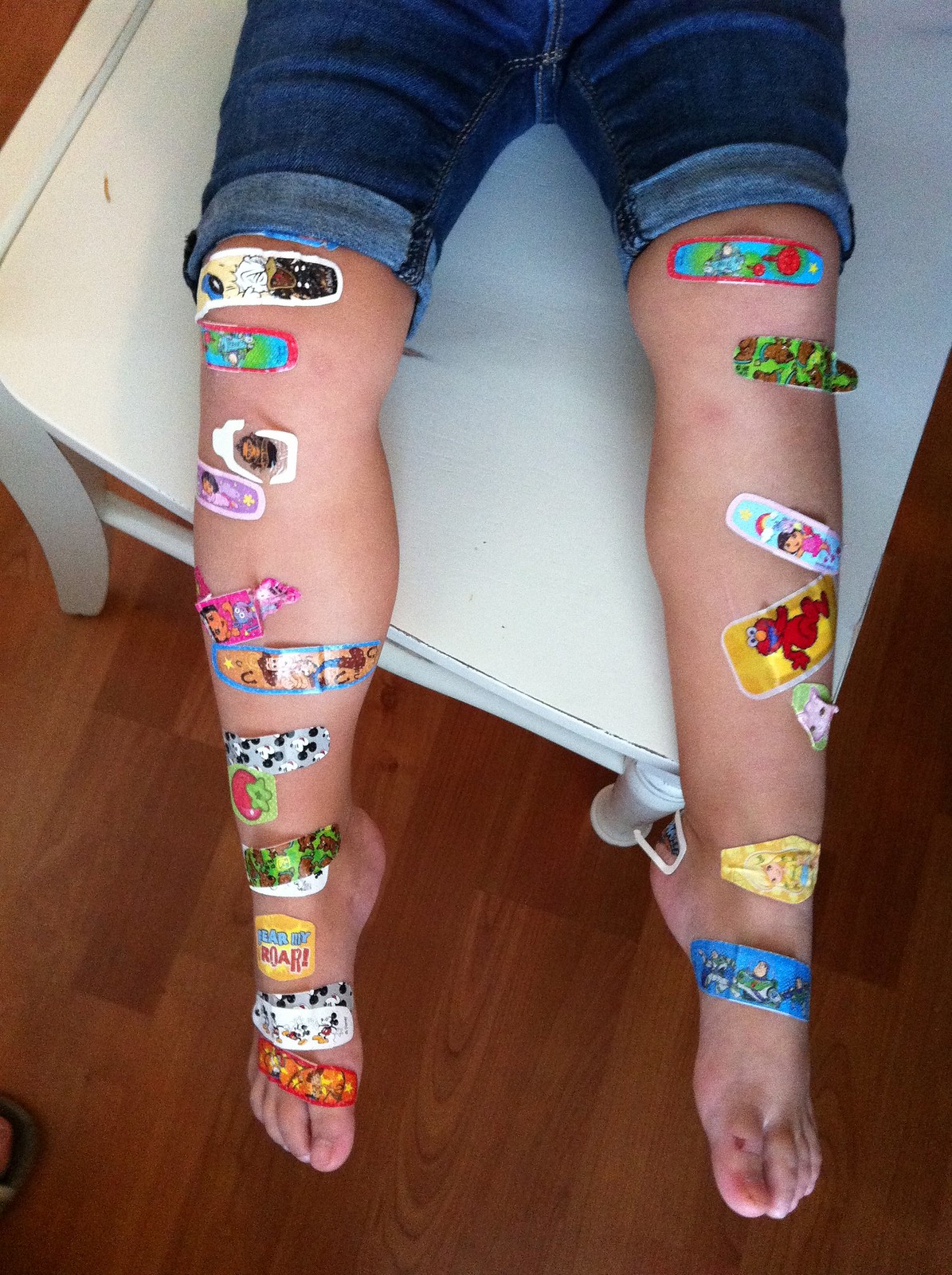The photograph depicts the legs of a person reclining on a white surface—either an office bed or a chair—above a brown hardwood floor. They are wearing dark blue jean shorts that have been rolled up at the thighs, and their bare legs, from the knees down to the toes, are covered in an eclectic assortment of colorful band-aids. The band-aids vary in design and size, featuring characters like Dora the Explorer, Elmo, Scooby-Doo, Woody from Toy Story, and more. Some band-aids are long and thin, others are large patches, and there are also little square ones. Notably, there is even one on the right heel. The person's legs appear stubby and short, contrasting with their longer feet and toes. The vibrant collage of band-aids includes themed designs, such as one with "Fear My Roar," another with tomatoes, and several with characters from Looney Tunes and Bratz. The overall image is a whimsical, colorful display of band-aids on the person's legs.